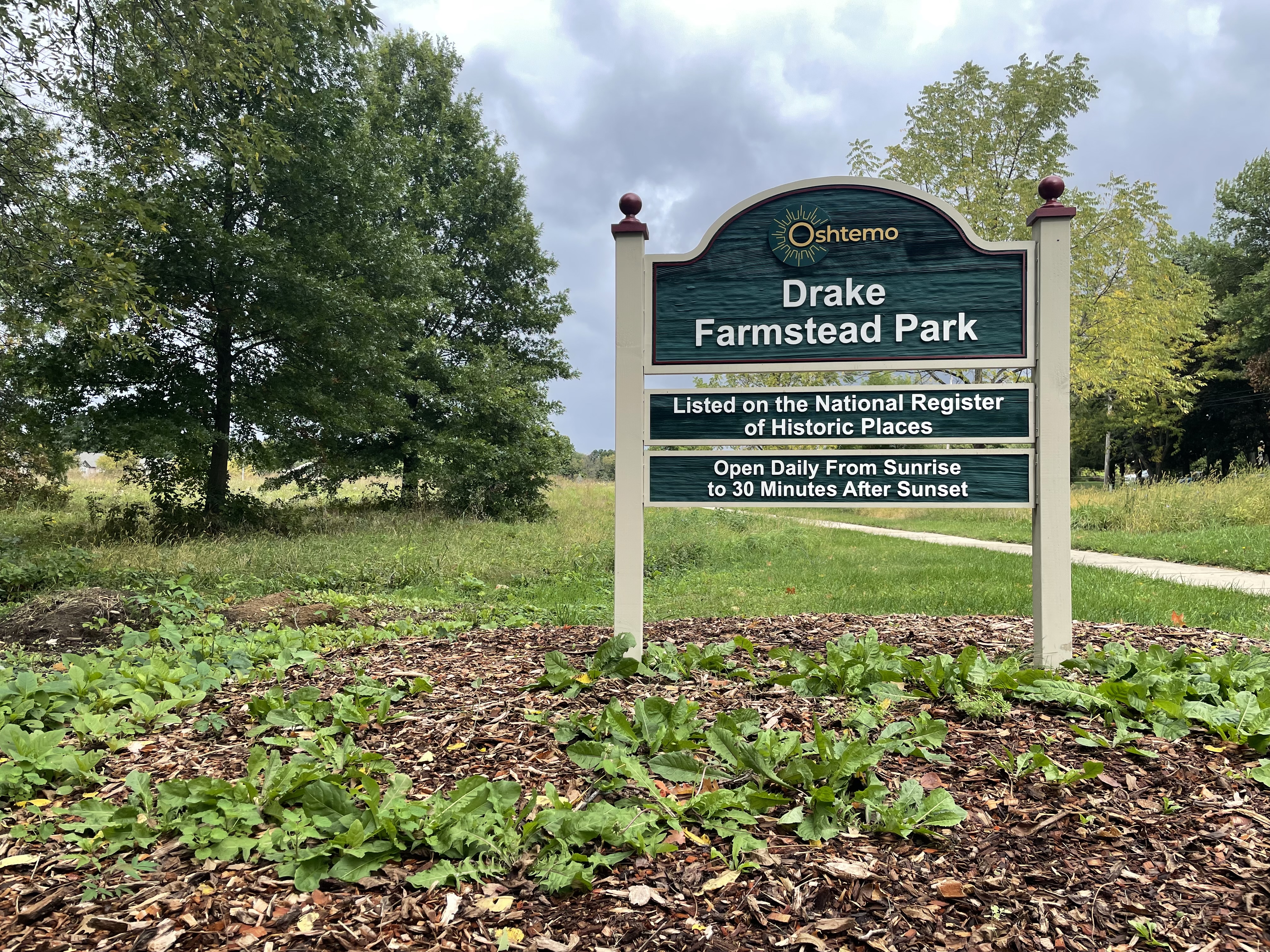In the foreground of the photograph, a rustic sign reads "Drake Farmstead Park," proudly listed on the National Register of Historic Places, with opening hours from sunrise to 30 minutes after sunset. The sign is set amidst a small flower bed, currently unplanted but covered in mulch with some weeds sprouting through. The middle ground reveals a grassy area with more weeds and a partially visible white concrete path on the left. In the background, an array of deciduous trees and overgrown grass frame the scene, while a pathway meanders into the distance. The overcast sky above is filled with grey clouds, hinting at an impending storm. The overall palette is a blend of green, yellow, and brown, lending a natural and somewhat untamed feel to the park setting.